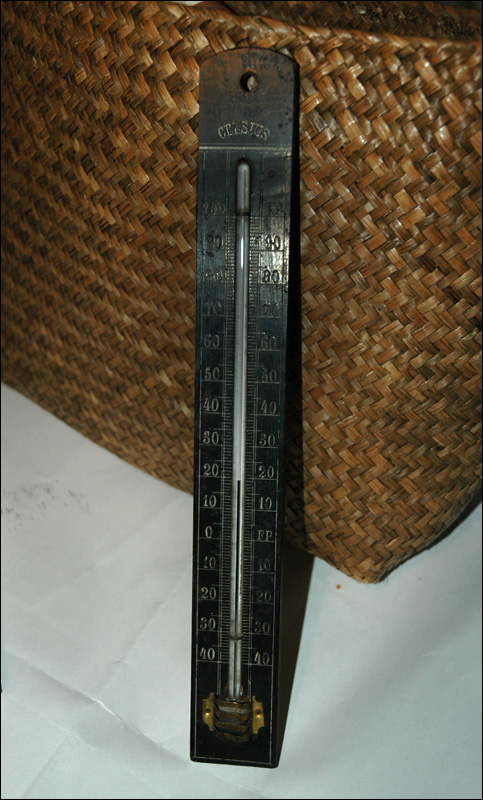This photograph features an antique-style thermometer prominently positioned at the center. The thermometer is encased in a tall, rectangular wooden frame with a dark, possibly painted finish. The wood is intricately crafted, featuring a cut-out section that snugly fits the thermometer. The graduated scales of the thermometer, marked with corresponding numbers in Celsius, are displayed on both the left and right sides of the instrument. These numerical indicators are identical on both sides, lending a symmetrical appearance.

Above the scales, the word "Celsius" is clearly labeled, signifying the unit of measurement. The thermometer is leaning against a wicker basket that occupies the upper half of the frame. The wicker basket, with its natural brown hues, contrasts against the dark wood of the thermometer. At the bottom of the image lies a folded white sheet, likely made of paper. This sheet is partially beneath both the wicker basket and the thermometer, forming the base of the composition. Overall, the photograph captures a rustic and homely scene with a focus on the vintage thermometer's detailed craftsmanship and setting.